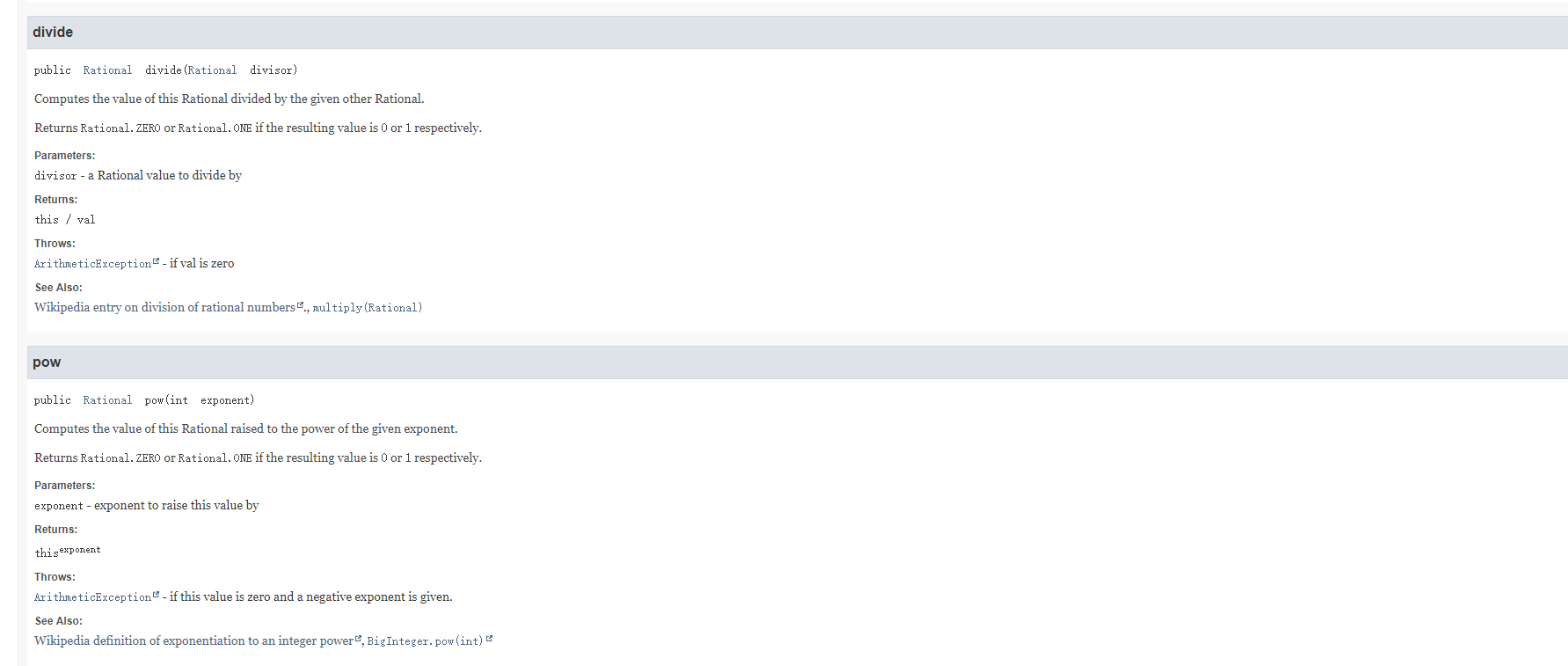This image displays a partial section of a website, as viewed from a laptop. The captured section lacks a bottom border, adding to its fragmentary appearance. The top left corner prominently features the word "divide" in bold, starting with a lowercase 'd'. This text is set against a grey banner background. Bordering this banner are very light grey lines forming a partial border along the top and left sides of the image, with no borders on the right and bottom edges.

Beneath "divide," there are several lines of text, although the wording is difficult to decipher. The first word appears to be "public," and further along, it seems to include the words "divide" and "compete." Positioned at the bottom of this section is the phrase "see also Wikipedia," followed by a space.

The next highlighted section begins with "POW," written in black font and starting with a lowercase 'p'. This term is also set against a grey banner, mirroring the style used for "divide." The "POW" section contains more lines of text, comparable to the ones under "divide." At the end of these lines, it also directs readers to "see also wiki, Wikipedia."